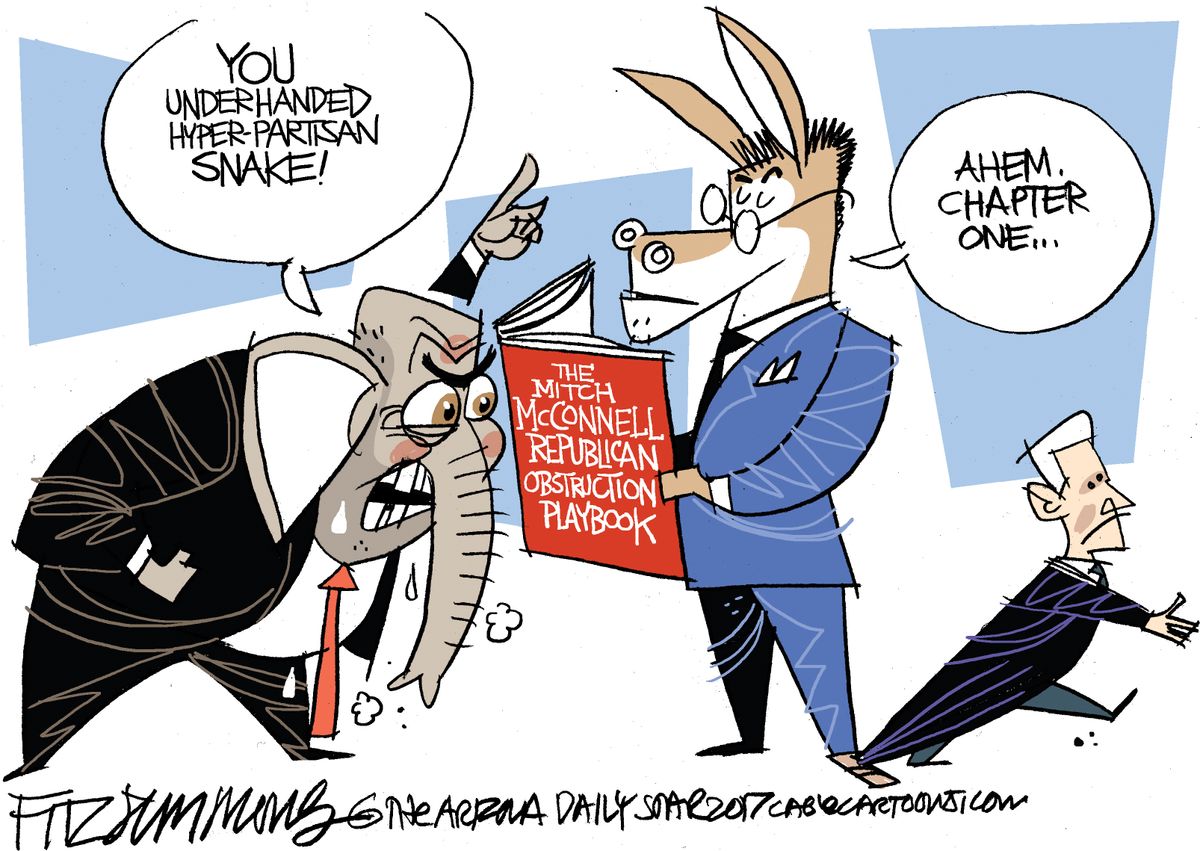This image is a political one-page comic strip resembling those found in newspapers, featuring an elephant and a donkey, emblematic of the Republican and Democratic parties, respectively. The angry elephant, sweating with red cheeks and forehead, is dressed in a black suit with a reddish tie, and is pointing while exclaiming, "You underhanded hyper-partisan snake" in a word bubble. On the right, the composed donkey, dressed in a crisp blue suit with black and blue pants and glasses, is reading from a red book titled "The Mitch McConnell Republican Obstruction Playbook" in white letters, and responds with, "Ahem, Chapter 1." The donkey has its foot on the back of a character resembling Mitch McConnell, identified by his gray hair and black suit, who appears beneath them with a displeased expression. At the bottom right corner, partially legible text seems to include the artist's signature, potentially "Fitzsimmons," and mentions a website, "dailysomethingcartoons.com."